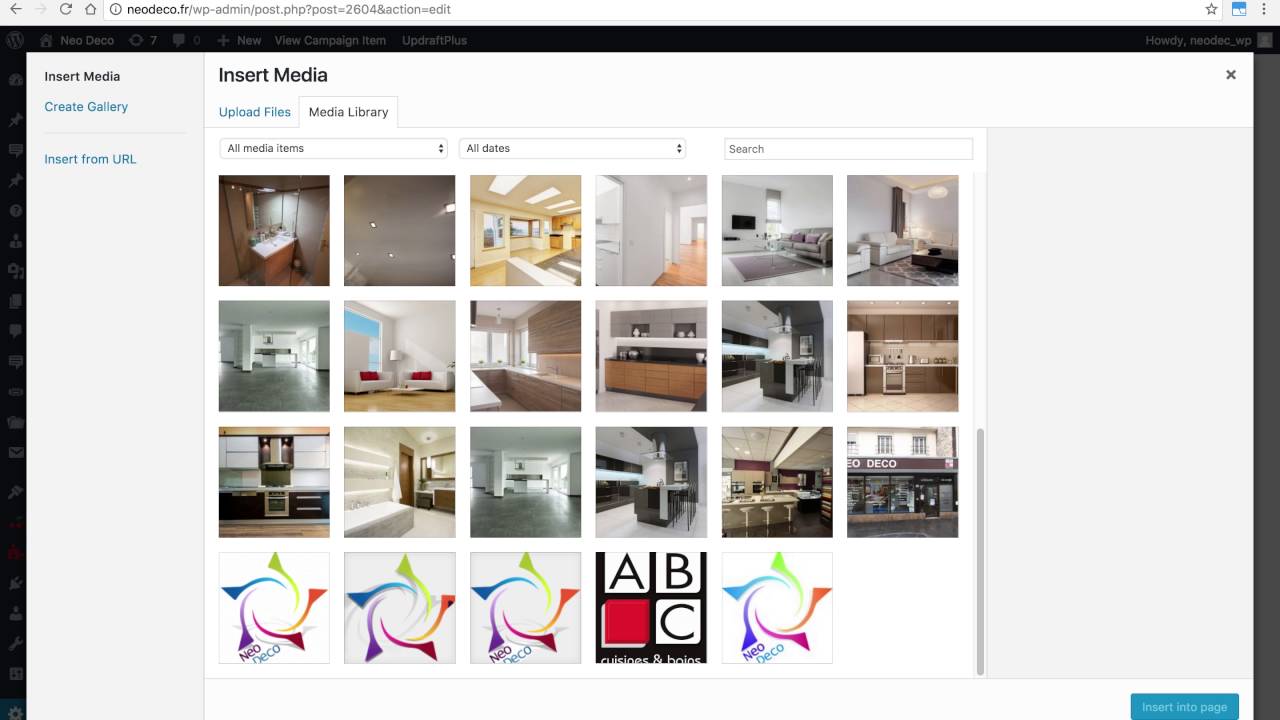The image captures a web interface that appears to be a media uploader or library within a content management system. At the top of the web page, there is a thin gray toolbar featuring standard browser navigation icons including a left arrow, a right arrow, a refresh button, and a home button. Adjacent to these icons, there is a white search or address bar displaying the website's URL.

Surrounding the main content area, there is a prominent black border that spans the entire left side, top, and right side of the interface. On the left section within this black border, there is a gray sidebar with text elements. The sidebar includes a black label that reads "Insert Media," followed by a blue link that says "Create Gallery," and another black label below it that says "Insert from URL."

The main content area of the page is set against a white background. At the top, it has a bold black heading that reads "Insert Media." Just below this heading, there is a blue link labeled "Upload Files" and a subsequent black heading that says "Media Library." Encased within a highlighted box, the interface presumably allows for user interaction.

Beneath this section, there is a lower panel featuring several options: a drop-down menu labeled "All Media Items," another drop-down menu labeled "All Dates," and a search field. This section displays a grid of image thumbnails, arranged six across and four down. However, the last row contains only five items. The images showcase various indoor settings, including kitchens, bathrooms, and living rooms.